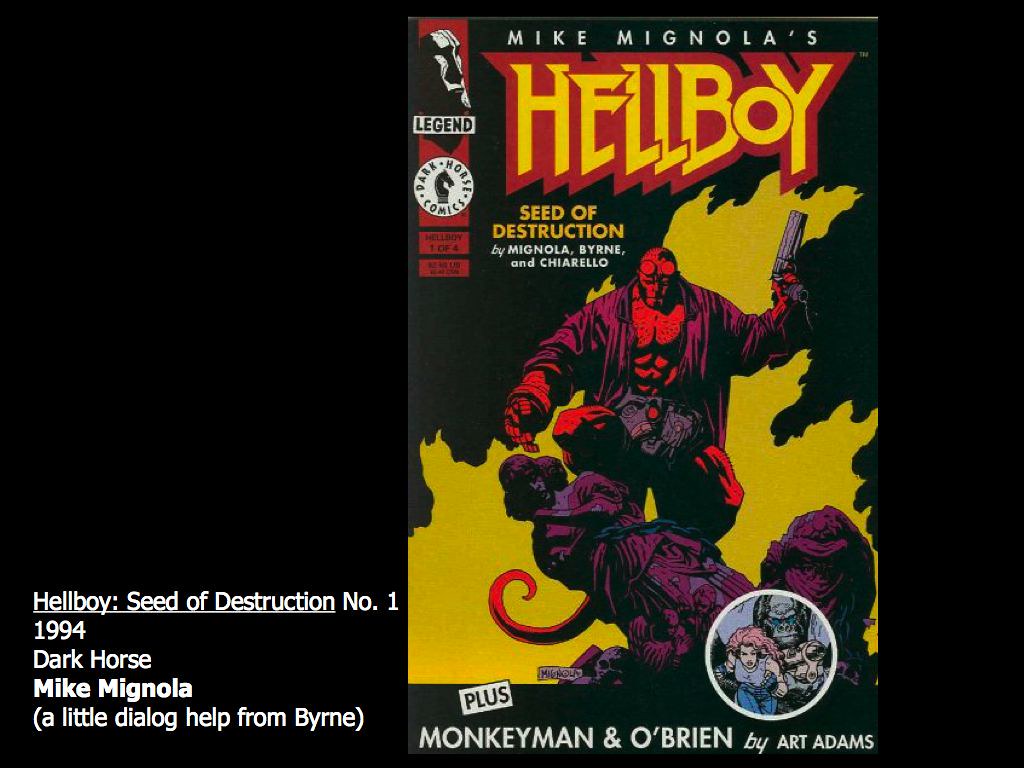The image features a comic book cover with a black background. Dominating the design, the title "Hellboy" is prominently displayed in bold yellow and red letters. Beside this, it reads "Seed of Destruction," also in yellow. Below, creator details are provided: "by Mike Mignola with a little dialogue help from John Byrne." The character of Hellboy, a large red figure, is illustrated front and center, clad in a purple cloak and wielding a gun. Additional text highlights "Hellboy Seed of Destruction No. 1, 1994," published by Dark Horse Comics. At the bottom, the cover also teases another feature: "plus Monkey Man and O'Brien by Art Adams."